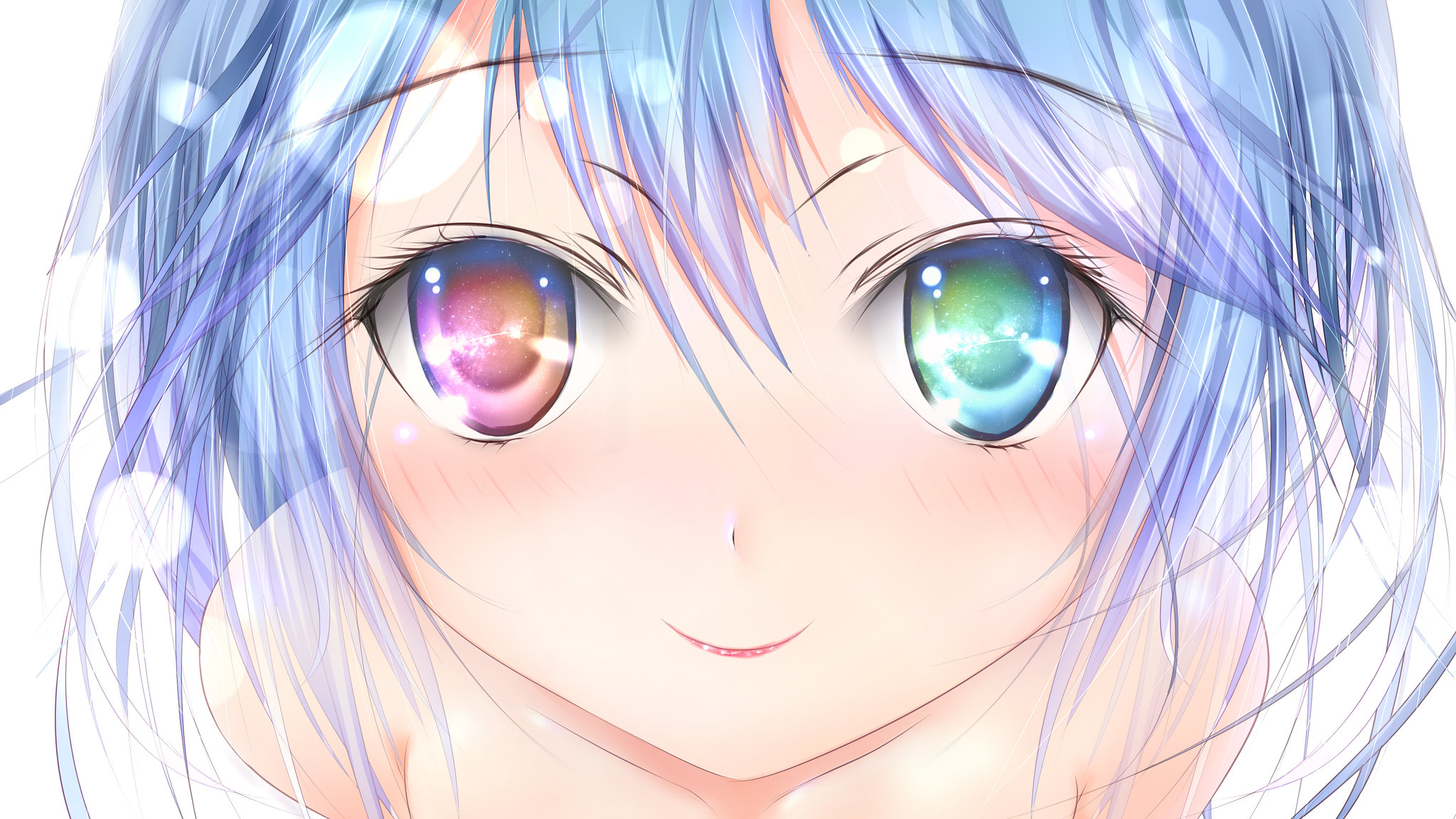This image is a detailed close-up drawing of an anime-style young woman, filling most of the screen with her head and shoulders. She has distinctive, wispy hair that is a mix of various shades of blue and purple, reaching chin-length with thin, wispy bangs gently falling between wide-set, large eyes. Her left eye is a unique blend of pink, blue, and purple hues, while her right eye transitions from green to blue with a brownish pupil. Her nose is minimalistic, depicted as a tiny dot, and she has a subtle, thin smile on her red lips. Her eyebrows are extremely thin, concentrated toward the center of her face, and her eyelashes are also quite delicate. Surrounding her head are small bubbles, particularly noticeable on her right side, and she appears to be staring directly ahead. The girl's skin is a creamy caucasian tone, and she is either against a white background or wearing a white, strapless piece of clothing that gracefully falls off her shoulders.